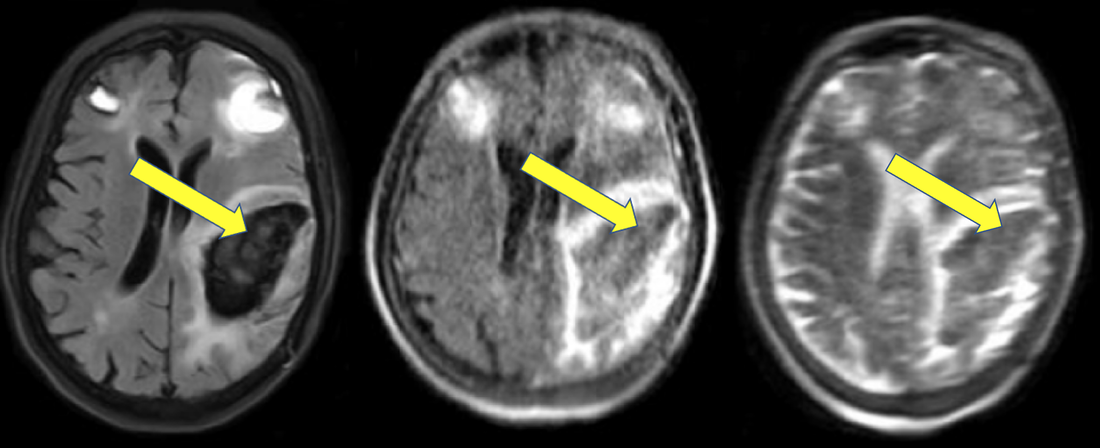The image showcases three separate brain scans, arranged side by side from left to right against a pure black background, forming a horizontally long rectangle. Each scan, displaying the top of a person's head, indicates a specific point of interest marked by a prominent yellow arrow. These arrows are oriented obliquely down from left to right, with their tips pointing towards a region in the bottom right of each scan. The brain is most distinctly detailed in the leftmost scan, showing clear delineation of the left and right hemispheres and revealing a dark pocket on the right side of the brain. The middle scan highlights this pocket with a bright white border, while the rightmost scan, although fuzzier and less clear, still displays a slightly less bright white border around the same area. These variations suggest the use of different scanning techniques to capture various details of the brain. The yellow arrows evidently point out a particular region of concern or interest in each image.